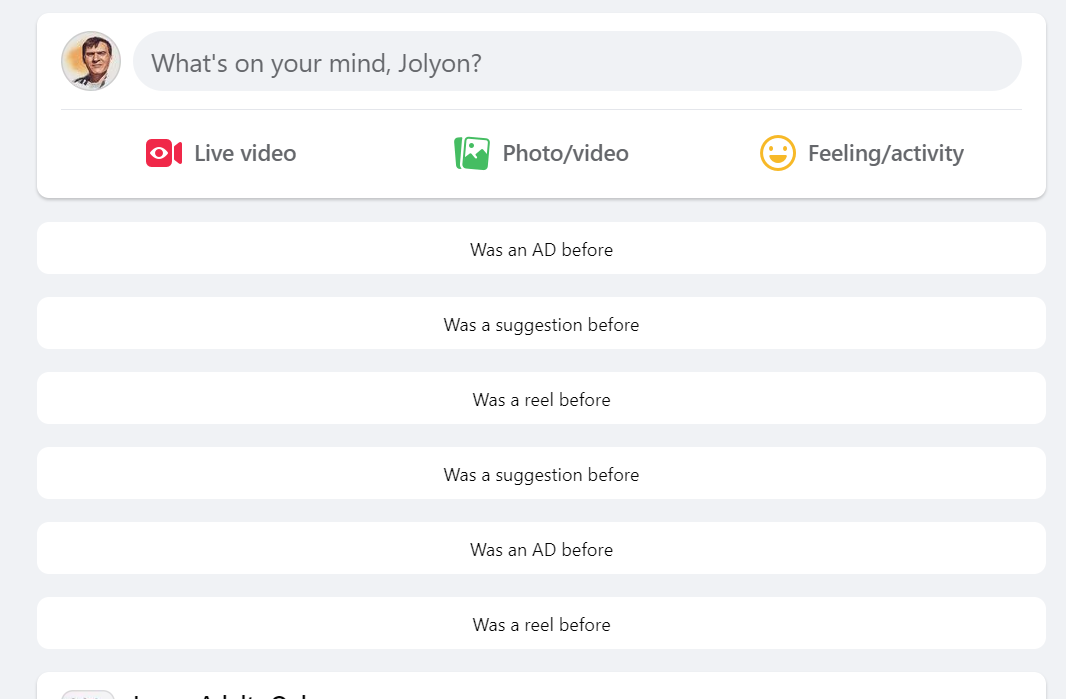The image appears to be a screen capture from a social media website. It has a white background with a profile picture of a man on one side. The man has brunette hair and a prominent nose, and there is an orange object behind his head. Directly beneath the profile picture is a text box with the placeholder "What's on your mind, Jolyon?" (J-o-l-y-o-n).

Below the text box, there are three icons arranged horizontally:
1. A red video camera icon with an eye, labeled "Live Video."
2. A green photo icon with a mountain, labeled "Photo/Video."
3. A gold smiley face icon, labeled "Feeling/Activity."

Further down, there are six white boxes with gray font. Each box contains text such as "was an ad," "was a suggestion," and "was a reel," repeated in various combinations. These texts are enclosed within white bubbles, separated by thin gray lines.

At the bottom of the image, there is a partial view of another box with some black text, although the text is not fully visible and unreadable.

The image itself is of clear quality and is framed by a thin gray border around its entirety.